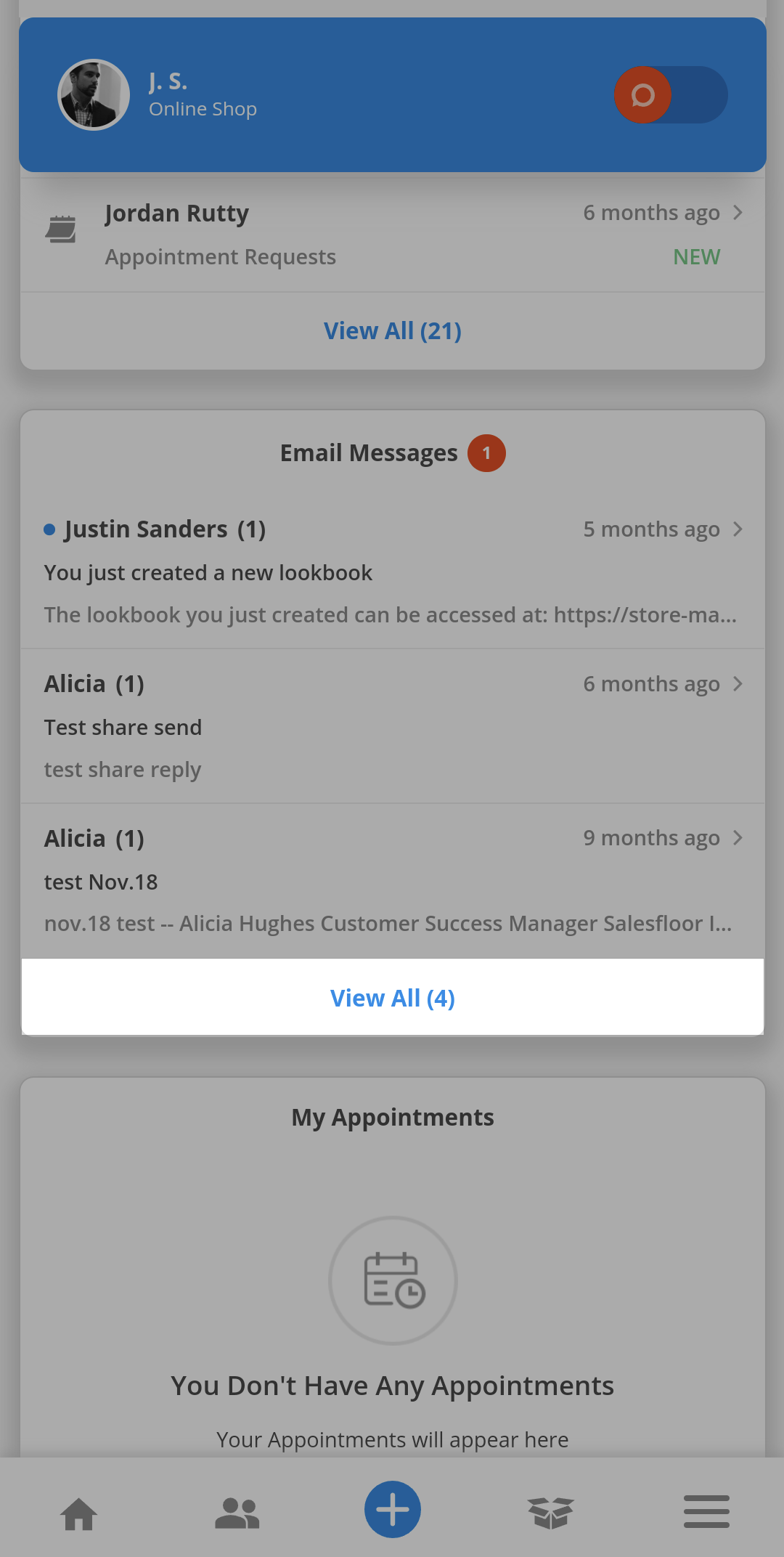The mobile app screenshot displays various information about a shop with a semi-transparent gray overlay, highlighting a central white box labeled "View All Four," which appears to be hovering over the rest of the content. At the top of the screen, a blue header features a profile image of a man in a suit, sporting a thin beard and a checkered shirt. To the left of the profile image, the text "J.S. Online Shop" is displayed, accompanied by a red button placed to the left of a grayed-out oval.

Beneath this section, the text "Jordan Ruddy appointment requests six months ago, new, view all 21" is visible, suggesting recent and past appointment requests. Further down, a section titled "Email Messages" contains a red circle with the number "1" indicating an unread message.

The email messages section includes:
- Justin Sanders: "You created a new lookbook. The lookbook you just created can be accessed at https://store-ma."
- Alicia: Multiple entries such as "test, share, send, test, share, supply," "test November 18th," and "test Alicia Hughes customer service manager sales floor."

Finally, the "My Appointments" section states, "You don't have any appointments" with the note that appointments will appear in this section when they are scheduled. At the bottom of the screen, there are icons depicting a home, a person, a plus sign, and an open box, presumably for navigation within the app.